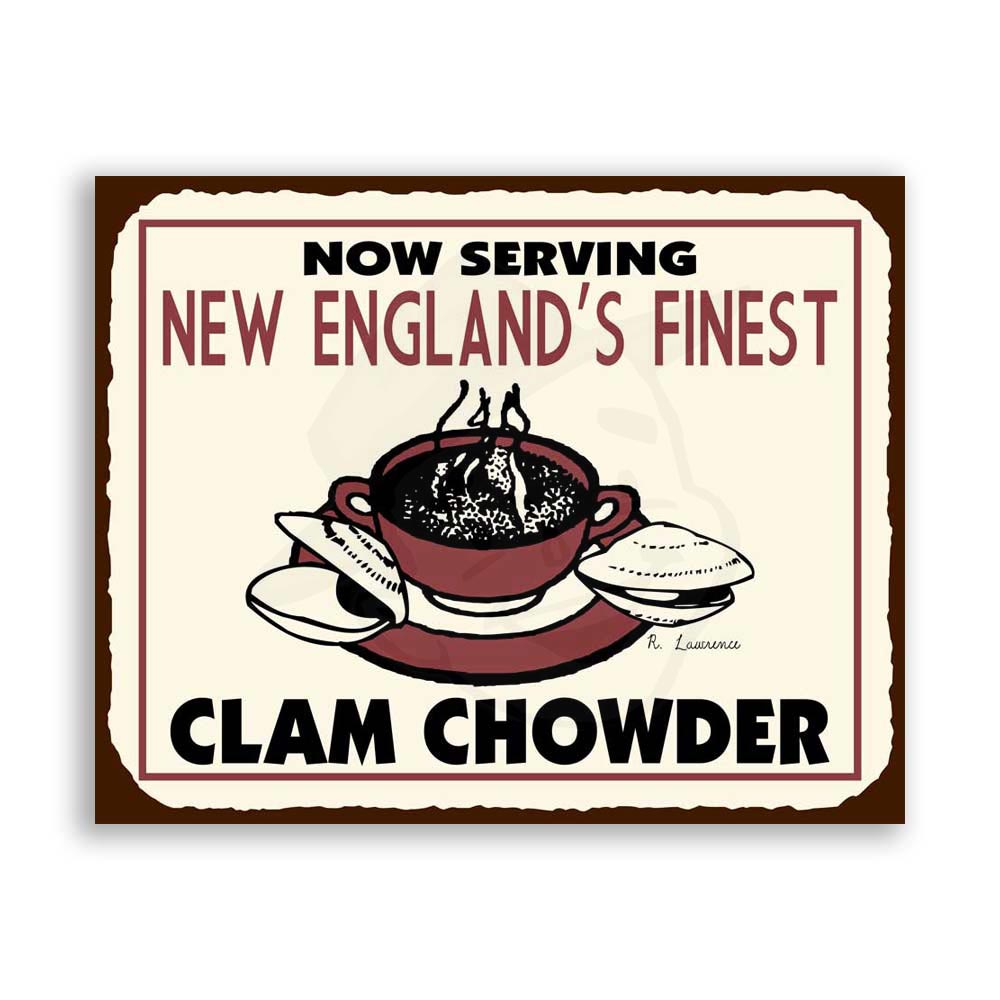The image depicts a digital sign for a restaurant, featuring a promotional ad for clam chowder. The overall background is a stark white, providing a clean and clear canvas. Centered on this background is a light tannish horizontal panel, bordered by a rich brown frame. Inside this brown-bordered panel, there's a vivid red rectangular border that frames the central design elements.

At the top of the sign, in bold black uppercase letters, it states, “NOW SERVING.” Below this, in a thinner and slightly taller maroon font, it proclaims, “New England's Finest.” The focal point of the sign is a meticulously drawn image of a maroon soup bowl with handles, emitting gentle wisps of steam to illustrate its warmth. This bowl rests on a matching maroon and white plate. Complementing the bowl are two clams placed symmetrically on either side of the plate—one clam is open, revealing its insides, while the other remains closed, noted by its white exterior with delicate black etchings adding detail.

Completing the advertisement, centered at the bottom of the sign, is the bold text “CLAM CHOWDER,” also in black but in a larger font, mirroring the style of the “NOW SERVING” text above. Framing the entire composition is a thin burgundy square border, ensuring the elements are enclosed in a cohesive and appealing manner. This sign, with its detailed illustrations and thoughtful typography, captures the essence of a charming restaurant or diner’s advertisement for their New England clam chowder.